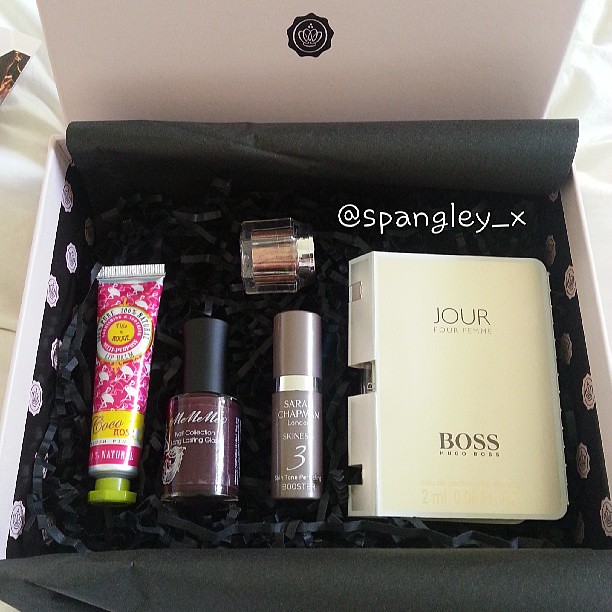This detailed color photograph captures a neatly arranged gift box of beauty and care products, evidently designed for a woman. The box is open, revealing five distinct items nestled on a bed of crinkled, black paper mimicking straw, complemented by black tissue paper that was initially meant to cover the items. Inside, from left to right, there's a metal tube of all-natural lip balm in a pink and yellow design. Adjacent to it lies a glass container of dark burgundy nail polish. Next is a tube of lipstick labeled "Sarah Chapman, No. 3." Above that sits a tiny, decorative glass jar, likely containing cream or lotion. Dominating the right side of the box is a sample of Hugo Boss fragrances, encased in a large, white square container. The white cardboard box, with its sturdy composition, rests on a white bed sheet, suggesting the photograph was taken from above by the photographer standing over the bed.